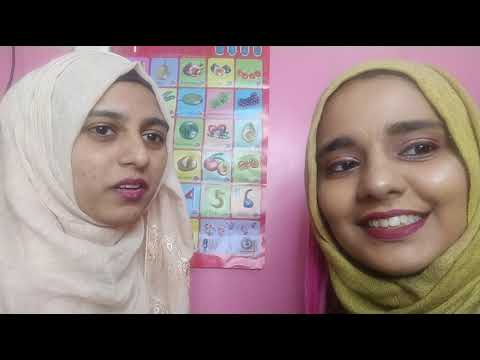In this indoor, horizontally rectangular, full-color photograph, two Muslim women stand in front of a pink wall with a poster displaying various shapes, food items, and numbers, including a visible four, five, and six. The image is framed with black borders on the top and bottom, but not on the sides. Both women wear hijabs, partially revealing their dark hair. The woman on the left is adorned in a cream-colored headscarf, has dark eyebrows, and wears purplish lipstick, with her mouth slightly open. The woman on the right smiles warmly, dressed in a yellow headscarf with burgundy-red lipstick. Both are facing the camera but gazing towards the right side of the image. We see them from just above the shoulders, capturing primarily their heads and part of their upper torsos.